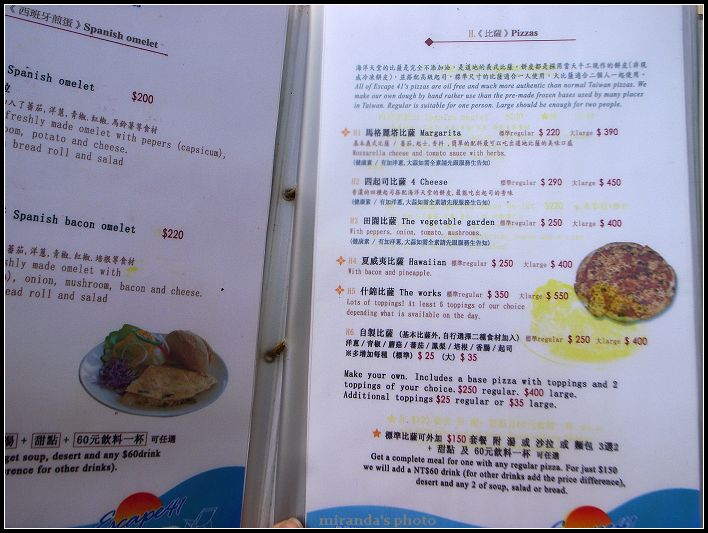This vibrant color photograph captures a close-up view of a restaurant menu laid open to two pages. The menu itself is pristine white with a hint of blue at the bottom, styled in a wave-like design, and branded with the name "Miranda's" in distinctive lettering. 

The left page of the menu features both Chinese characters and English descriptions. Prominently displayed is the "English-Spanish Omelette," described in multiple languages, priced at $200. This freshly made omelette includes peppers, potatoes, and cheese, and is served with a bread roll and salad. Additionally, the menu lists various other omelettes such as the "Spanish Bacon Omelette," which is slightly more expensive at $220. 

The right page also contains Chinese writing and introduces the pizza offerings, accompanied by a vivid image of a pizza. This section lists several pizza varieties: "Margarita" at $220, "Cheese" at $290, "Vegetable Garden" at $250, "Hawaiian" at $250, and "The Works" at $350. There's an option to create your own pizza, starting with a base and two toppings for $250. Additional information about other available pies is also provided. An inviting picture of an omelette graces the left page, enhancing the appeal of the dishes offered.